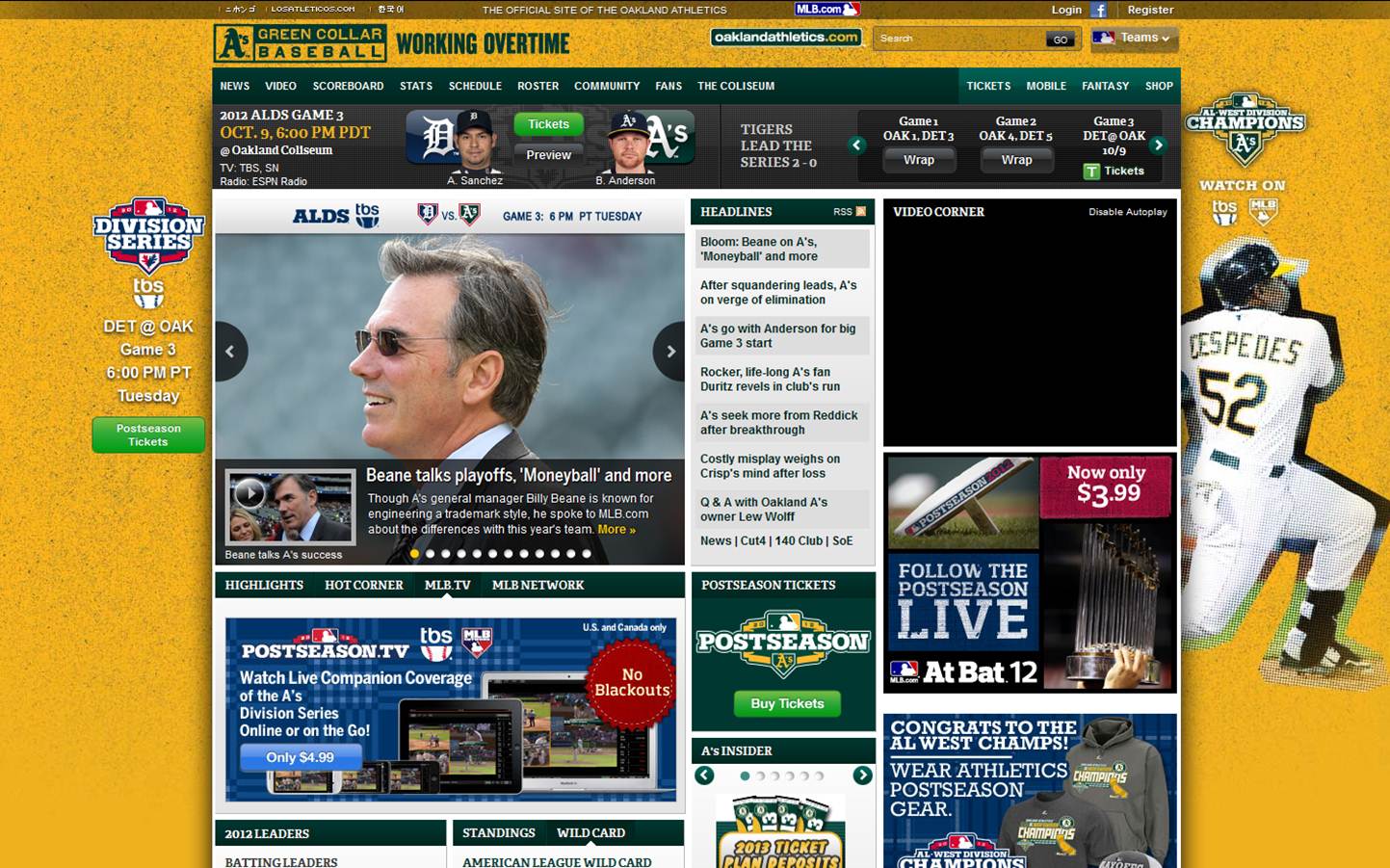The image is of a website, likely from the Oakland Athletics’ official site, as suggested by the URL and branding elements. In the upper left-hand corner, the logo of the Oakland Athletics is prominently displayed next to the phrase "Green Collar Baseball." Dominating the top center of the website is a banner featuring two baseball players, adding a dynamic and sporty feel to the page.

Below this banner, the site transitions into a section resembling a sports news portal. There's a visible headline that reads "Being Talks, Playoffs, Moneyball, and More," accompanied by a picture of a man looking towards the left side of the screen, suggesting an interview or a feature article. Additionally, there's a headline section and a video corner showcasing "Follow the Postseason Live," alongside mentions of "Postseason.TV," indicating a focus on live updates and video content related to ongoing playoff games. The site appears to be a comprehensive source for Oakland Athletics fans, offering news, interviews, and live updates.